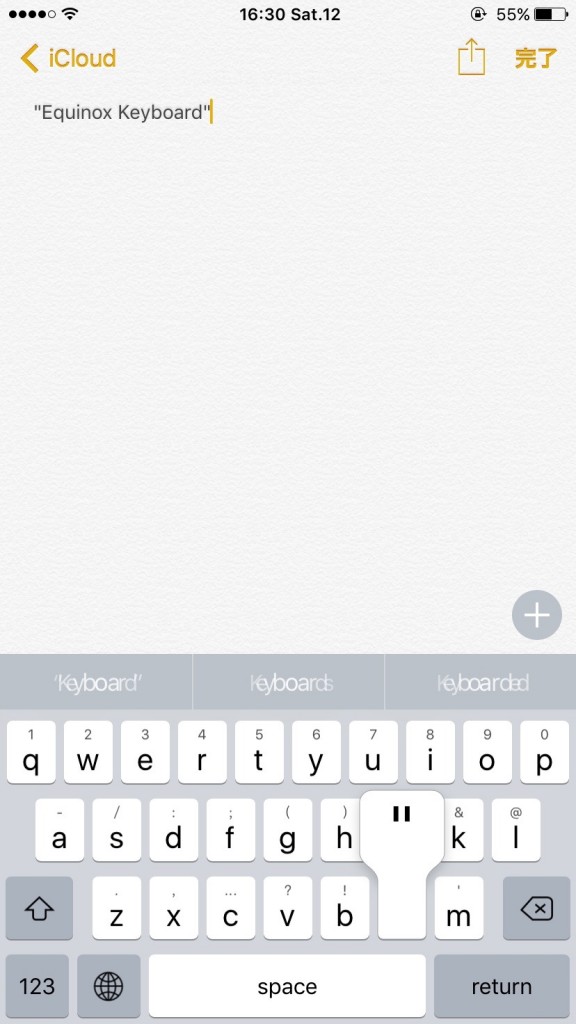The screenshot showcases someone's mobile phone interface, captured at precisely 16:30 on a Saturday, the 12th. The time is prominently displayed at the top center of the screen. To the right, the battery indicator shows 55% remaining power, while the signal strength indicator on the left displays five dots, with four filled in black, indicating strong signal reception. Adjacent to this is the Wi-Fi symbol, confirming connectivity.

Directly below, the screen displays the word "iCloud" with an open arrow pointing to the left. On the right side of this, there is oriental writing, the specifics of which are unknown. Below "iCloud," an icon that appears to be an orange fruit is visible.

Centered on the screen is the phrase "Equinox keyboard" in quotation marks, typed in black text with an orange vertical cursor blinking behind it. The rest of the display is a serene light blue background, devoid of any additional icons or text.

At the bottom of the screenshot, there is a mention of different keyboard options: "keyboard," followed by "ittyboard," and then "ittyboardd." The QWERTY keyboard is prominently displayed, with pronounced quotation marks situated between the "B" and "M" keys. Additional keys include "123" for numeric input, a small globe symbol for switching languages, a space bar labeled "space," and a "return" key for concluding text entries.